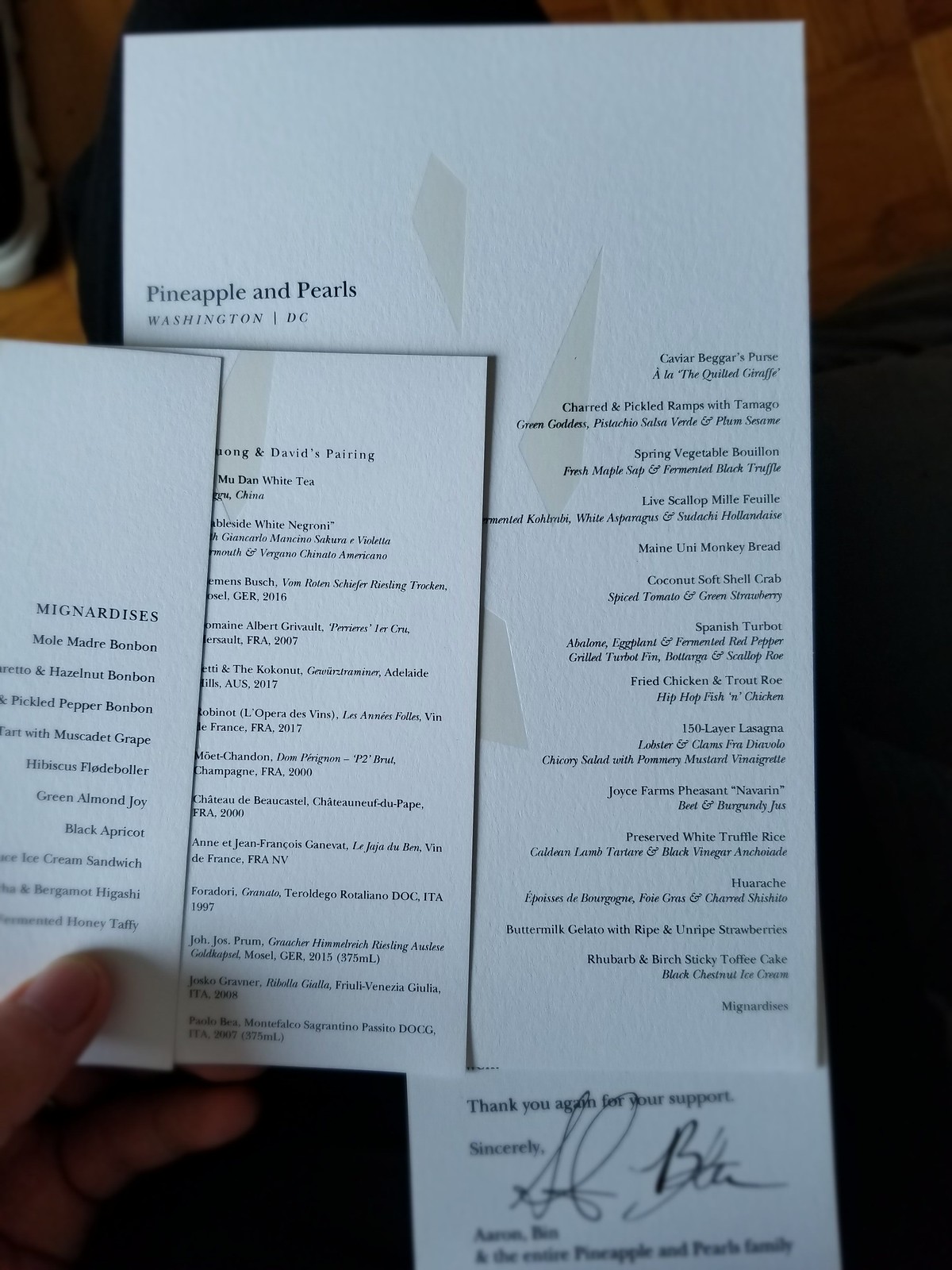This photograph captures a sophisticated menu from the upscale restaurant, Pineapple and Pearls, situated in Washington D.C. The menu comprises three overlapping sheets, each featuring an array of exotic dish names, without any prices listed. On the largest sheet, some of the highlighted dishes include Caviar Beggar's Purse, Charred and Pickled Ramps with Tamango, Spring Vegetable Bouillon, Live Scallop Mille-feuille, Maine Uni Monkey Bread, and Coconut Softshell Crab. The font used is very refined and elegant, adding to the menu's exclusivity.

A central list, written in an extremely small font, appears, while the left section features further items like Mole Madre Bon Bon, Hazelnut Bon Bon, and Pepper Bon Bon. The bottom part of the menu hints at a dessert list, including Green Almond Joy. At the very bottom, a courteous message reads, "Thank You Again for Your Support Sincerely."

The menu is printed on an off-white, light gray background, set against a darker backdrop. In the lower left corner of the photograph, a person's finger points towards what seems to be the dessert list, subtly emphasizing the luxurious and carefully curated dining experience offered by Pineapple and Pearls.